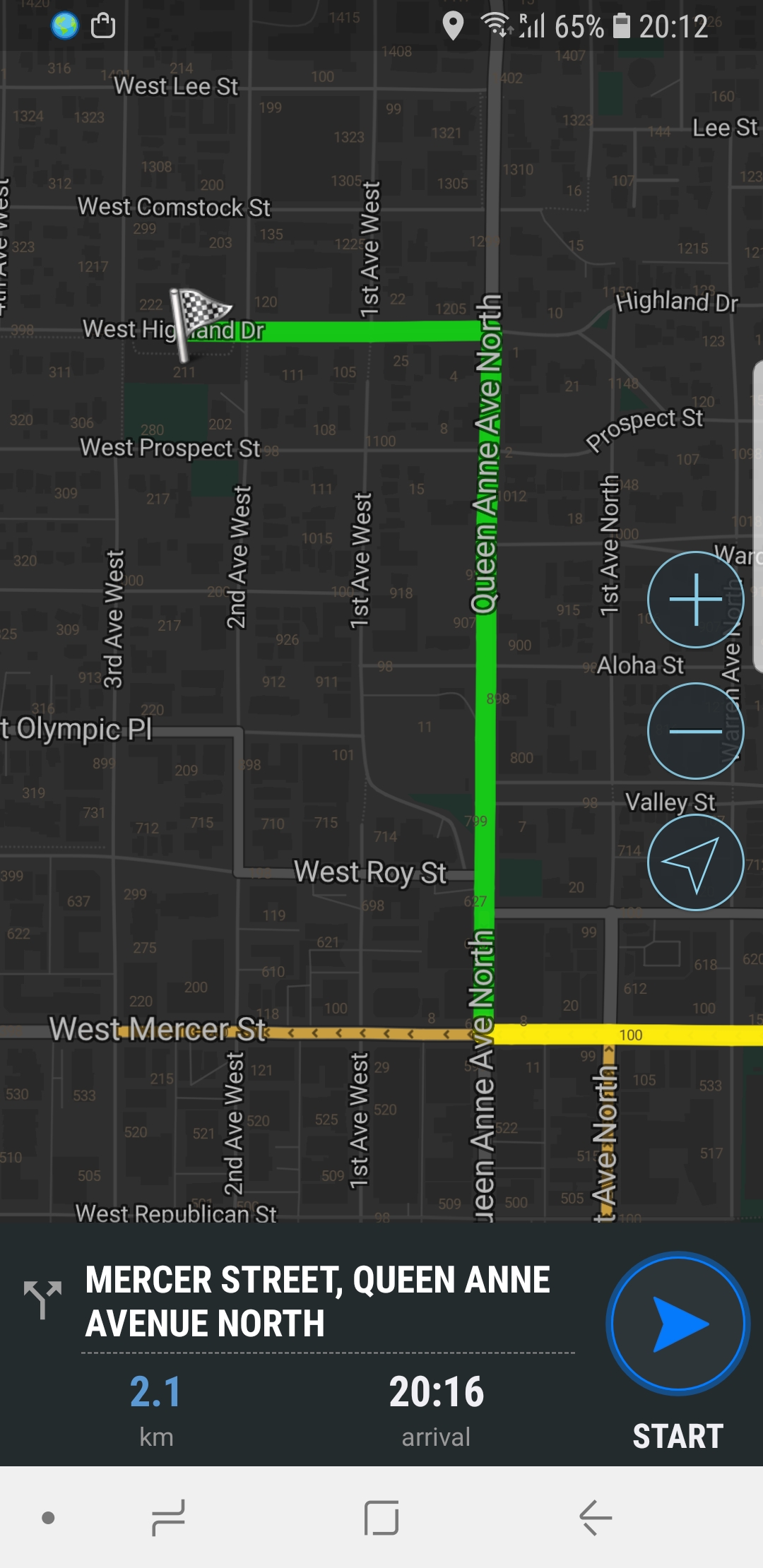Screenshot of a mobile GPS navigation app in dark mode, displaying a map of a specific route. The map features a green-highlighted road labeled West Highland that intersects with Queen Anne Avenue North. The route indicates a turn onto West Mercer Street, which is marked in yellow, suggesting traffic congestion. The journey covers a distance of 2.1 kilometers with an estimated arrival time of 20:16. The navigation interface includes a prominent blue start button, and the overall design adheres to a black-themed dark mode for reduced glare and visual comfort.